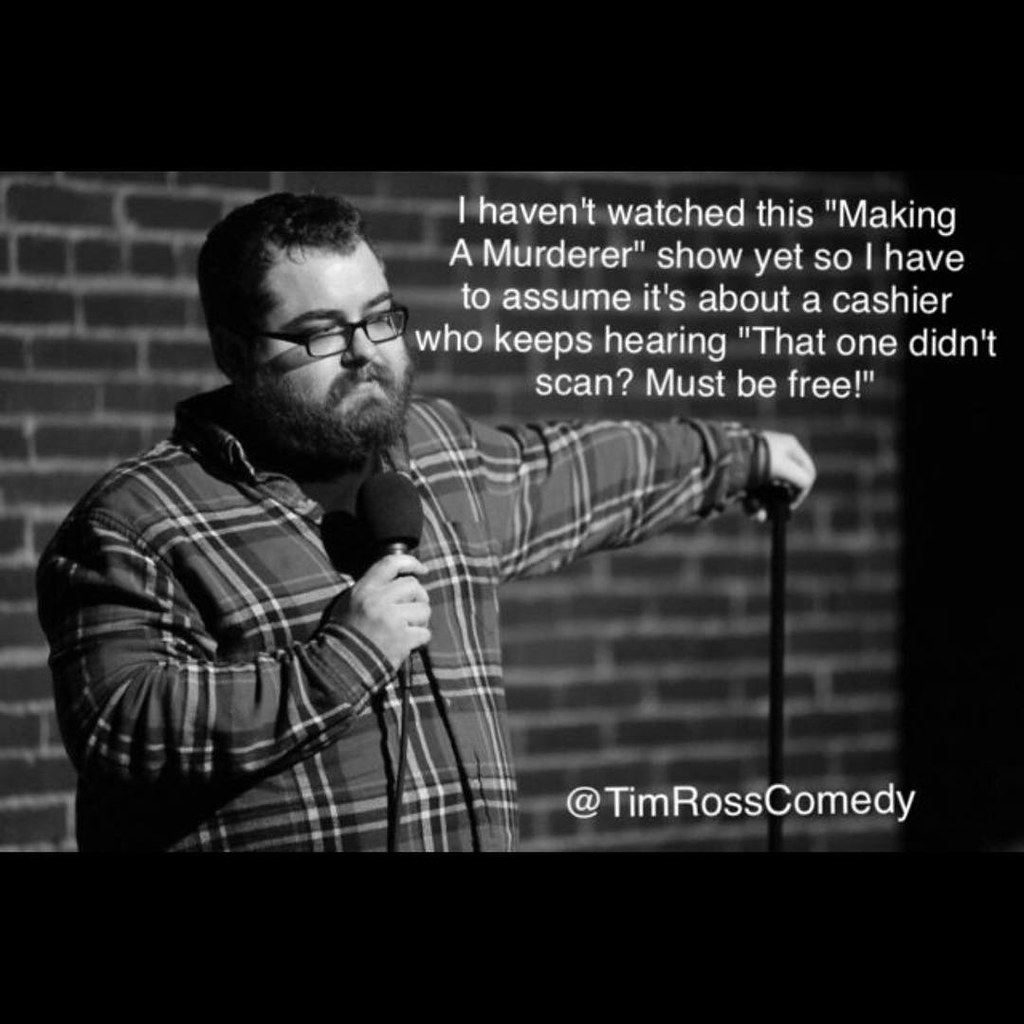The black-and-white photograph captures a bearded man standing on a stage, dressed in a long-sleeved plaid shirt and black-rimmed glasses. He holds a microphone in his right hand, while his left hand casually rests on a microphone stand. The stage features a brick wall as the backdrop, contributing to the stark, monochrome aesthetics. The image is framed by black borders at the top and bottom, enclosing a scene meticulously detailed yet devoid of any color. Superimposed at the top, white text reads, "I haven't watched this 'Making a Murderer' show yet, so I have to assume it's about a cashier who keeps hearing, 'That one didn't scan. Must be free.'" In the bottom right corner, further white text advises, "Follow me @TimRossComedy."